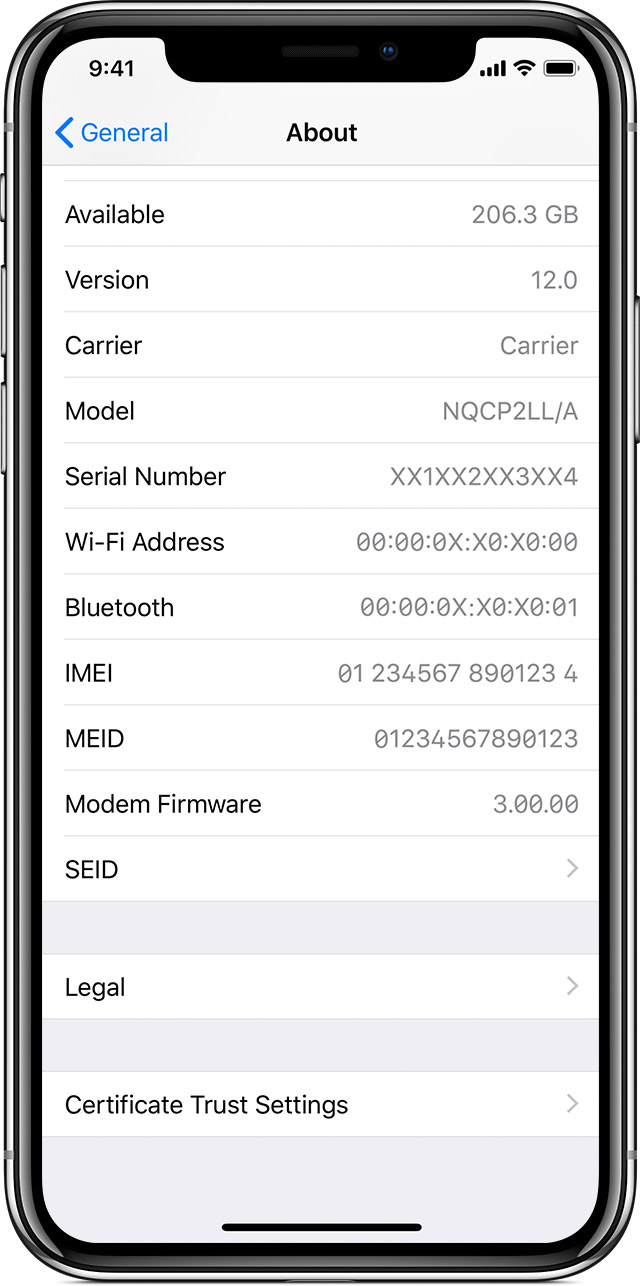**Descriptive Caption:**

The image showcases a meticulously designed CGI representation of an iPhone. The device features a prominent metal band around its edges, indicating the modern and sleek aesthetic typical of Apple's design language. The screen displays the "About" section of the phone's settings, which includes detailed system information.

At the top of the screen, the status bar reveals the time as 9:41, along with full signal bars, Wi-Fi connection, and battery. The interface exhibits a blue back button labeled "General" and centrally positioned text that reads "About." 

Key details provided on the screen include:
- Available storage: 206.3 GB
- iOS Version: 12.0
- Carrier: Displayed as "carrier"
- Model Number: NQCP2LL/A
- Serial Number: XX1XX2XX3XX4
- Wi-Fi Address: 00:00:0X:X0:X0:00
- Bluetooth Address: 00:00:0X:X0:X0:00
- IMEI and MEID: Placeholder numerical sequences 01 to 9 followed by 01 to 4 and 123 respectively
- Model Firmware: 3.00.00
- SEID and other information such as "Legal" and "Certificate Trust Settings" at the bottom of the screen

The intricate detail and placeholder text clearly indicate this image is a digital mock-up of the iPhone's "About" menu.